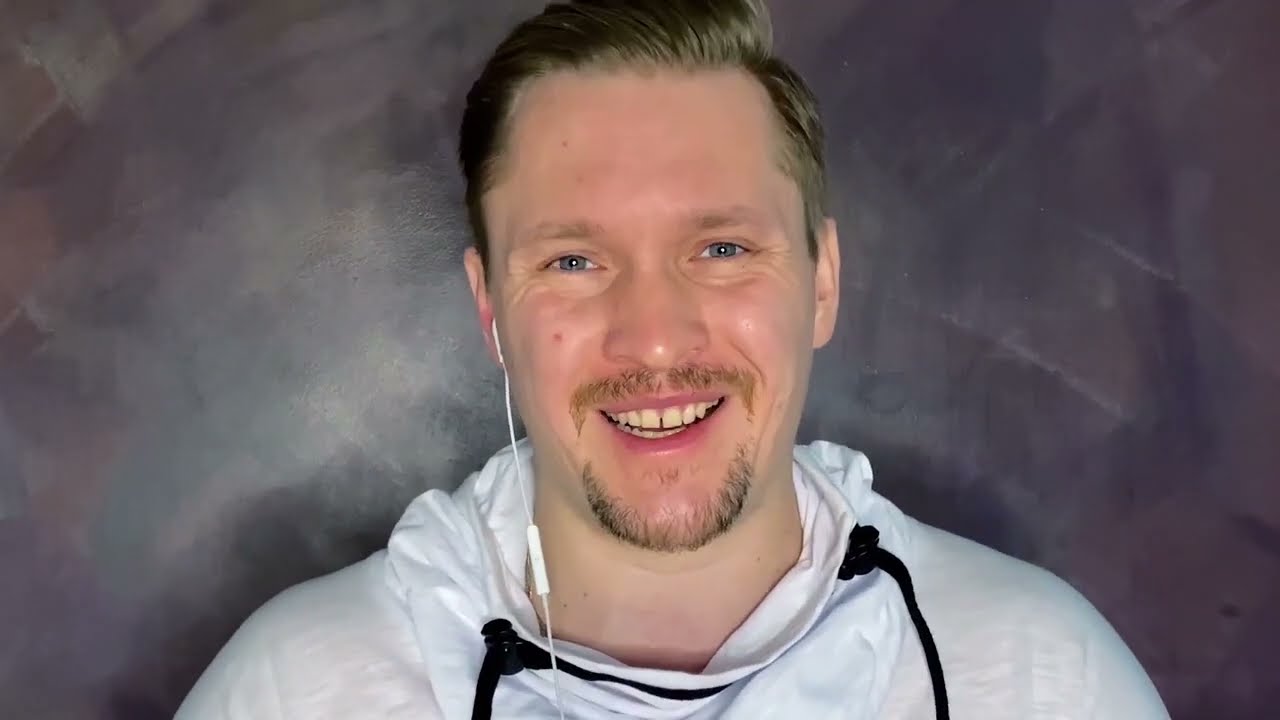This photograph features a man standing in front of a gray, mottled background that resembles the type used in photo studios. The background has varying shades of gray, somewhat reminiscent of a chalkboard with white smears. The man, who appears to be in his early 30s, is smiling and looking directly at the camera. He has short, light brown, or sandy brown hair and blue eyes. His facial hair includes a small mustache and a bit of beard. He is dressed in a white hoodie with black drawstrings, which are visible in front of him, and the hood is tucked behind. An earbud is hanging out of his left ear, suggesting he might be listening to music or on a call.